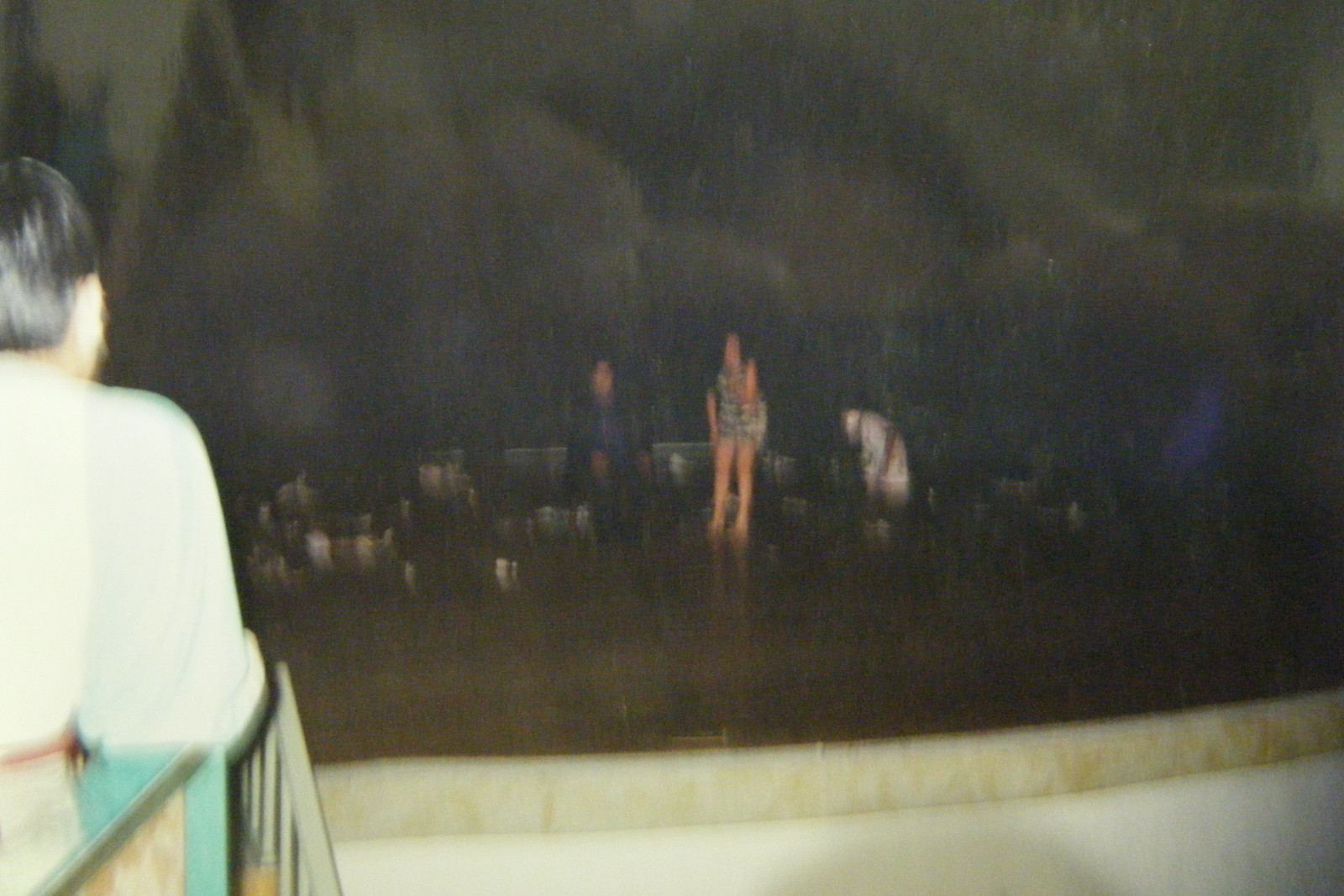This photograph captures a blurry nighttime scene, likely at a beach, obscured by light pollution and lens flare. In the foreground stands a person with short dark hair, dressed in light-colored clothing, precariously positioned on what appears to be metal stairs. The background reveals a group of individuals: one dressed in a white outfit with dark stripes, another entirely in white, and a third in blue, standing adjacent to the person in stripes. The overall lack of clarity renders the details indistinct, leaving much of the environment and activities ambiguous.